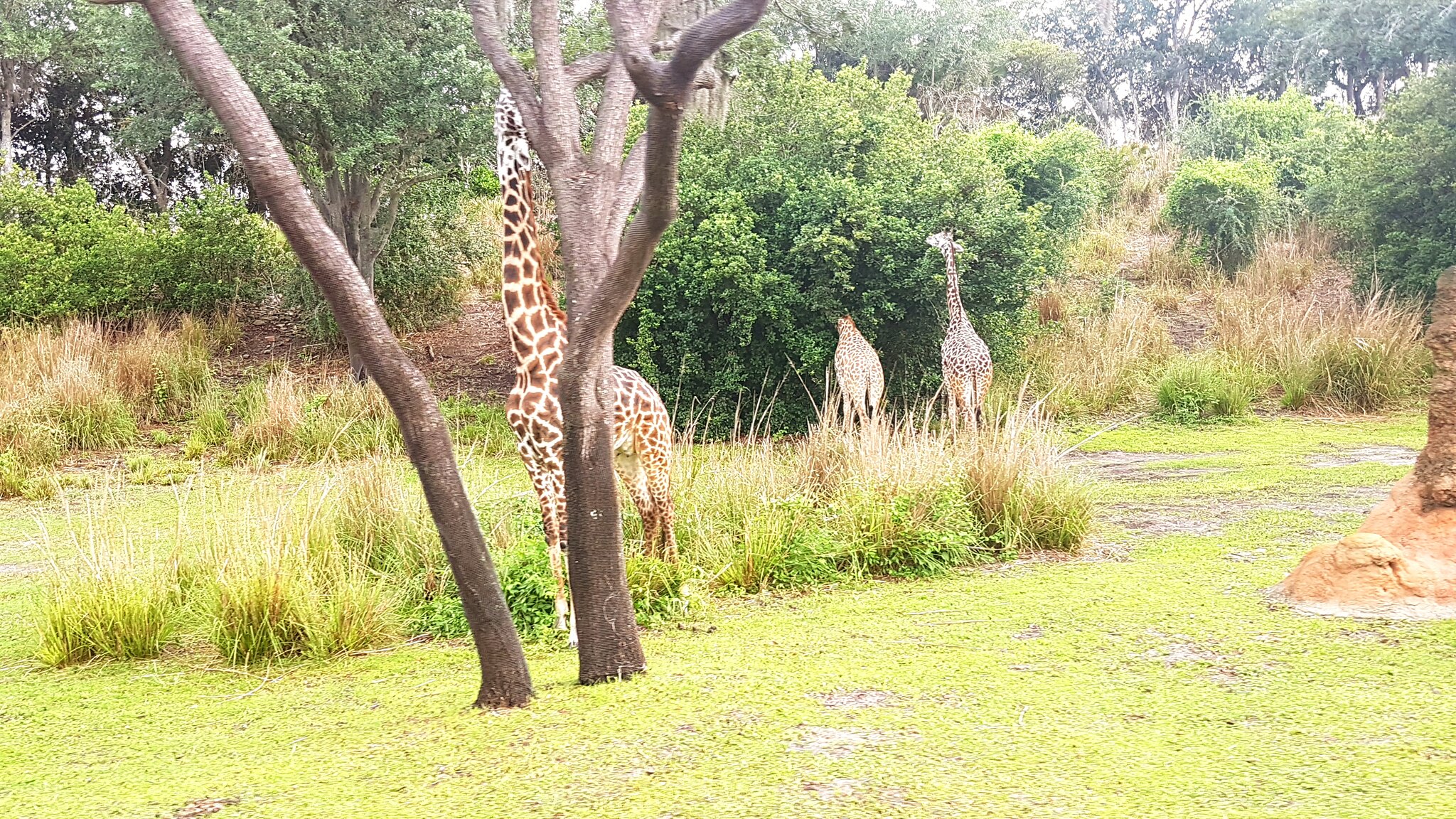The image depicts a vibrant African field, likely part of a safari or wildlife rescue area. The foreground showcases two prominent trees: one leaning diagonally to the left and the other standing straight with various upward-slanting branches. Nestled between these trees is a giraffe, seemingly reaching up for leaves, although its head is obscured by the tree. The landscape features a mix of short, light green grass and a distinctive patch of taller grass, roughly 2-3 feet wide and 10-12 feet long. Further in the background, a denser wooded area with lush greenery, bushes, and taller trees can be seen. The background also includes two more giraffes; one is browsing leaves with its neck extended, while the other bends down toward the base of a tree. An interesting detail at the right edge of the image is a brick-like structure with red mud beneath it, approximately 4-5 feet tall. The overall scene is bathed in sunlight, highlighting the varied shades of green and touches of beige from dried grasses, giving it a warm, natural ambiance.